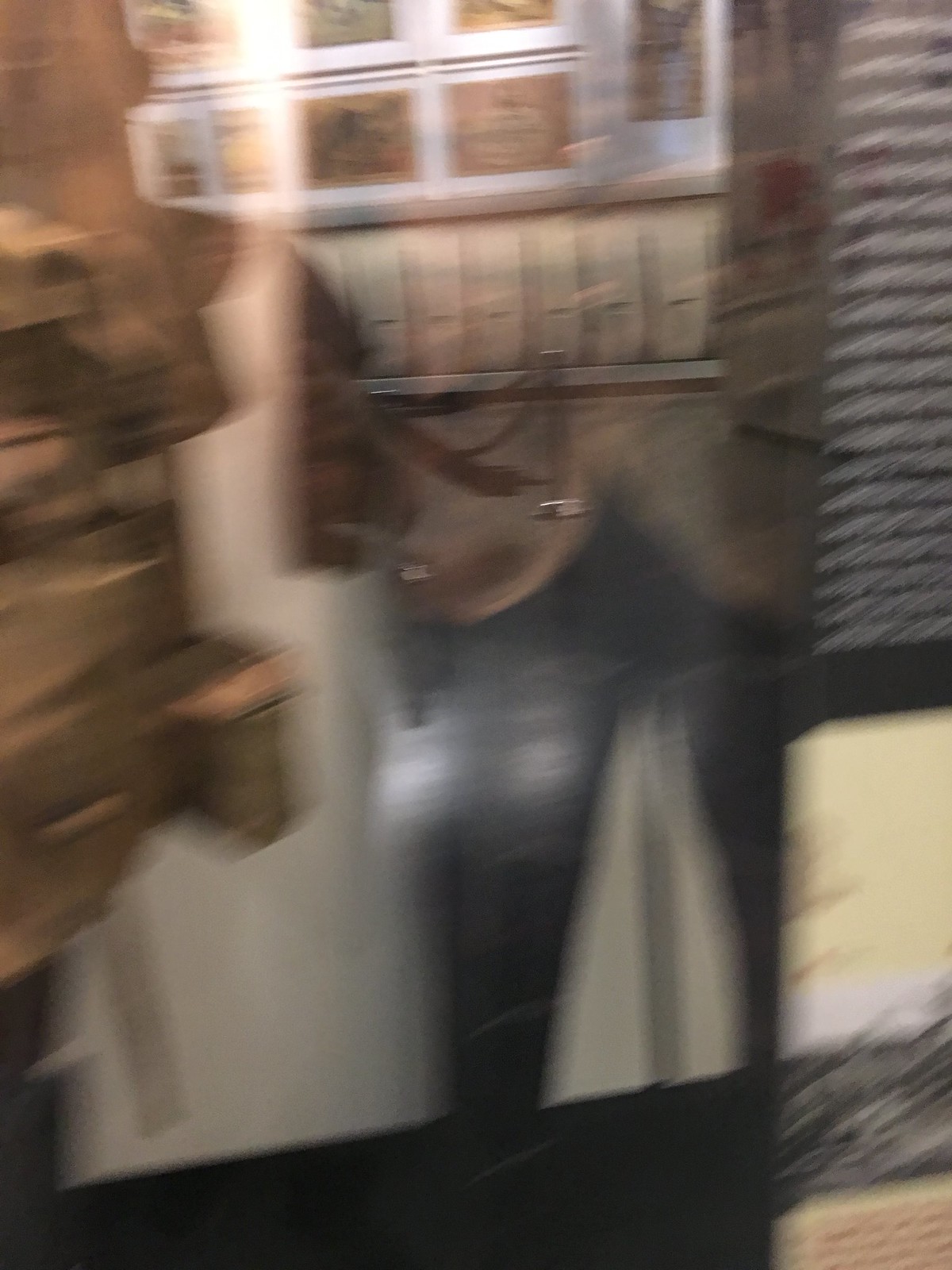In this highly abstract and blurred photograph, captured through a glass window, numerous reflections and motion blurs are present, making the details difficult to discern. The image shows a mix of inside and outside elements, creating a double-exposure effect. Dominating the foreground on the right are white horizontal lines resembling window blinds. Centrally, a silver pole with a rope, likely part of a velvet roping setup, is visible amid a background featuring several square pictures bordered in wood and white, hanging on a wall. On the left side, blurred brown and beige shapes, possibly resembling a stack of cardboard boxes or moving objects, further add to the complexity of the scene. Overall, the photograph is a chaotic blend of reflections, light distortions, and unclear objects, resulting in an almost abstract composition.